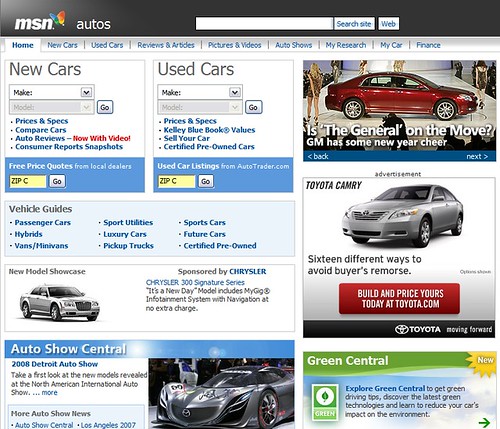This is a screenshot of the MSN Autos website, identifiable by the "MSN" label and the colorful butterfly logo in shades of orange, yellow, green, and blue located at the top left corner. The top right corner highlights the word "autos," indicating the automotive section of MSN. 

At the top of the page, a navigation bar provides access to multiple sections: Home (currently highlighted), New Cars, Used Cars, Reviews and Articles, Pictures and Videos, Auto Shows, My Research, My Car, and Finance.

Next to the MSN logo, there are options for exploring new and used cars. Users can select the make and model of a car and then click the "Go" button to search for available vehicles. Under the "New Cars" section, additional links include Prices and Specs, Compare Cars, Auto Reviews (now with video), Consumer Reports, and Snapshots. On the "Used Cars" side, links include Prices and Specs, Kelley Blue Book Values, Sell Your Car, and Certified Pre-Owned Cars. This comprehensive layout points to MSN Autos being a dedicated platform for car shopping and research.